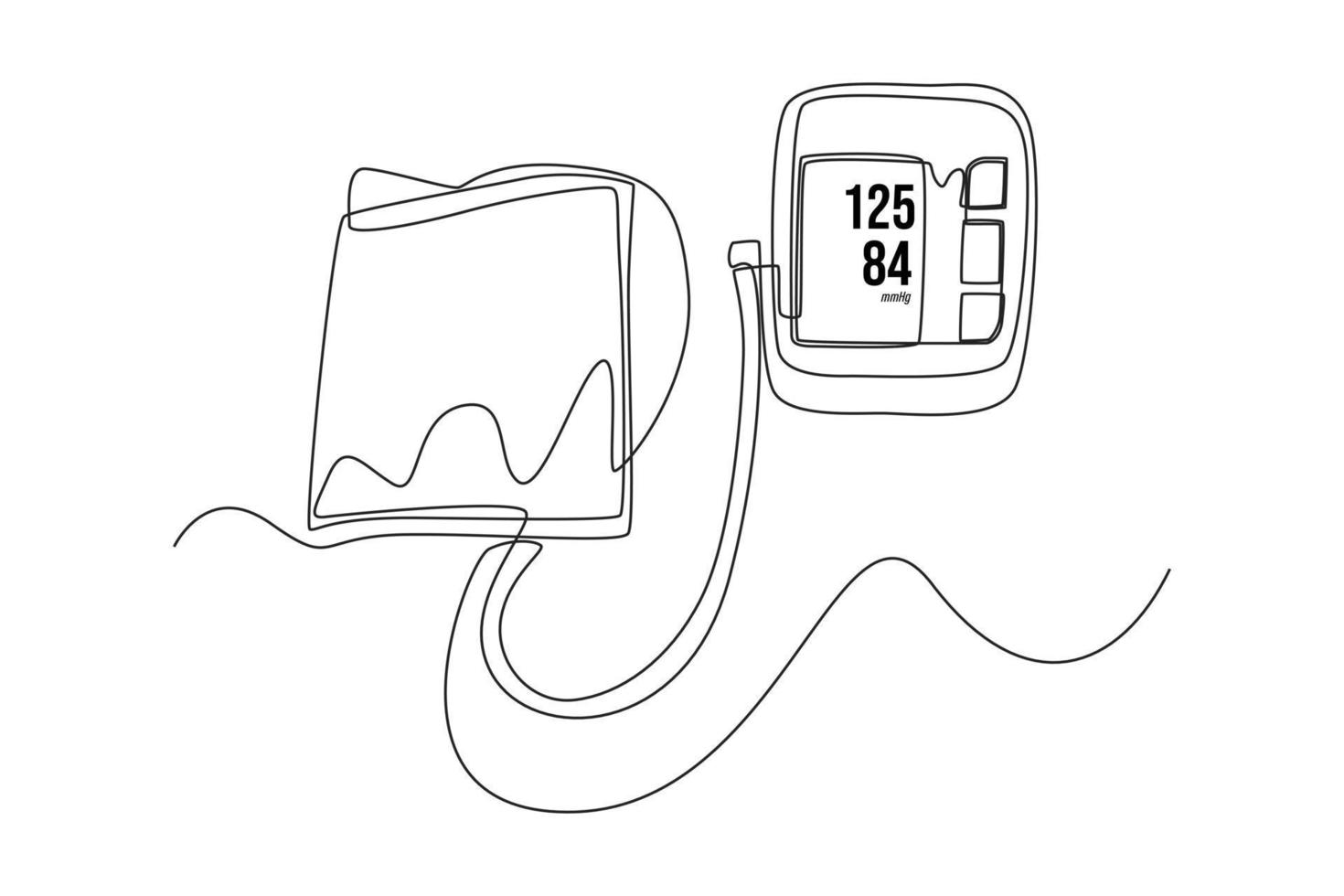This image is a crude, hand-drawn sketch in black on a white background, depicting a basic blood pressure monitor. The drawing features a simple rectangular meter displaying a blood pressure reading of 125/84, drawn with black lines on a white area. To the right of the meter, there are white squares trimmed in black. A cuff, similarly outlined in black and white, is attached to the meter by curved, squiggly tubing lines. The entire illustration appears rudimentary, resembling a doodle made with minimalistic pen strokes or even an etch-a-sketch, characterized by its simplicity and lack of color. No patient or additional components are depicted, leaving only the essential elements of the blood pressure monitoring device.